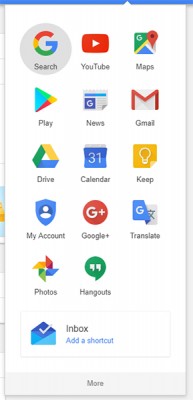This image is a screenshot of the application grid that pops up when accessing all available apps within a Google account. The background of the page is white, with a prominent dark blue horizontal line extending from left to right at the top of the image. The window appears to be superimposed on an email inbox within Gmail, indicated by some partially visible icons or folders on the left.

The grid features three columns of icons, organized into six rows. Each icon represents a different Google service:

- **First Row:** 
  - Top left: Multicolored "G" icon labeled "Search."
  - Center: Red play button icon labeled "YouTube."
  - Far right: Google Maps pin icon.

- **Second Row:** 
  - Left: Multicolored triangular play button icon labeled "Google Play."
  - Center: Newspaper icon labeled "Google News."
  - Far right: Red and white envelope icon labeled "Gmail."

- **Third Row:** 
  - Left: Triangular icon labeled "Google Drive."
  - Center: Calendar icon.
  - Far right: Yellow bulb icon labeled "Keep."

- **Fourth Row:**
  - Left: Icon labeled "My Account."
  - Center: Red circle icon with a white "G+" for the discontinued Google Plus.
  - Far right: Google Translate icon.

- **Fifth Row:**
  - Left: Pinwheel icon labeled "Photos."
  - Center: Green speech bubble icon with white quotation marks labeled "Hangouts."
  - Far right: Blue envelope with a white checkmark labeled "Inbox."

- **Sixth Row:**
  - Center: Text link labeled "More."

Overall, the image provides a comprehensive view of the various applications and services available through a Google account, showcasing popular options like Search, YouTube, Google Maps, and more.